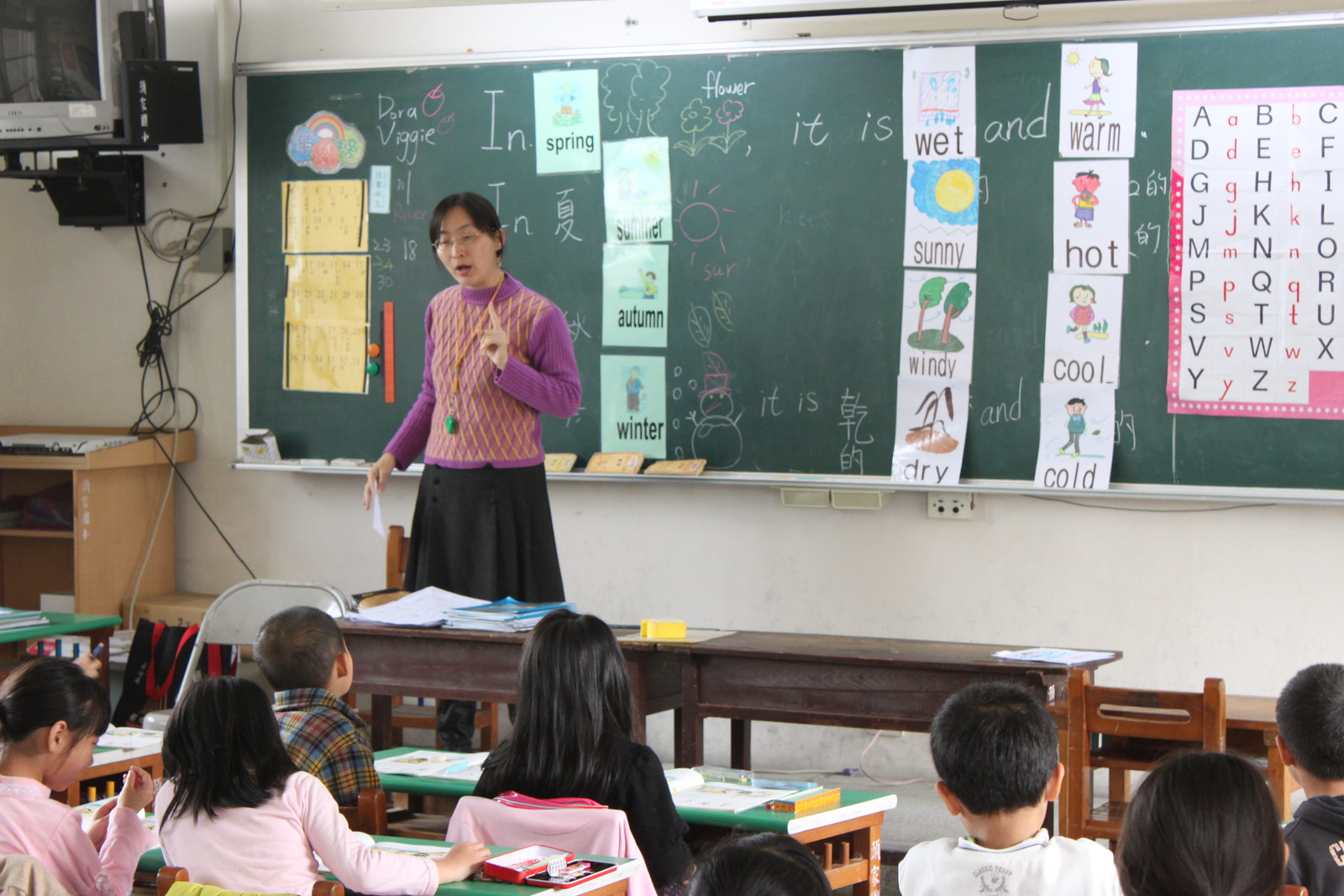In this detailed color photograph of a classroom, the viewer observes the scene from behind a group of students seated at small desks, looking toward their female teacher, who is standing at the front left side of the image. The teacher, with black hair and glasses, is dressed in a purple and yellow argyle sweater adorned with a green pendant, and a black skirt. She appears to be in mid-lecture, with her left arm raised, finger pointed up, potentially directing the students' attention.

The classroom features a large green chalkboard that spans horizontally behind the teacher. On the chalkboard, there are four colorful pieces of paper labeled with the seasons: spring, summer, autumn, and winter. Additionally, on the left third of the image next to the teacher, three yellow papers are taped to the board. The chalkboard also has various other writings related to weather, with terms like warm, hot, cool, cold, wet, sunny, windy, and dry displayed prominently. To the right side of the chalkboard, there is a poster of the English alphabet. In the upper left corner of the room, a TV monitor is mounted on the wall, enhancing the classroom's educational tools. The style of the image is photographic representationalism realism, capturing the dynamic and structured learning environment.